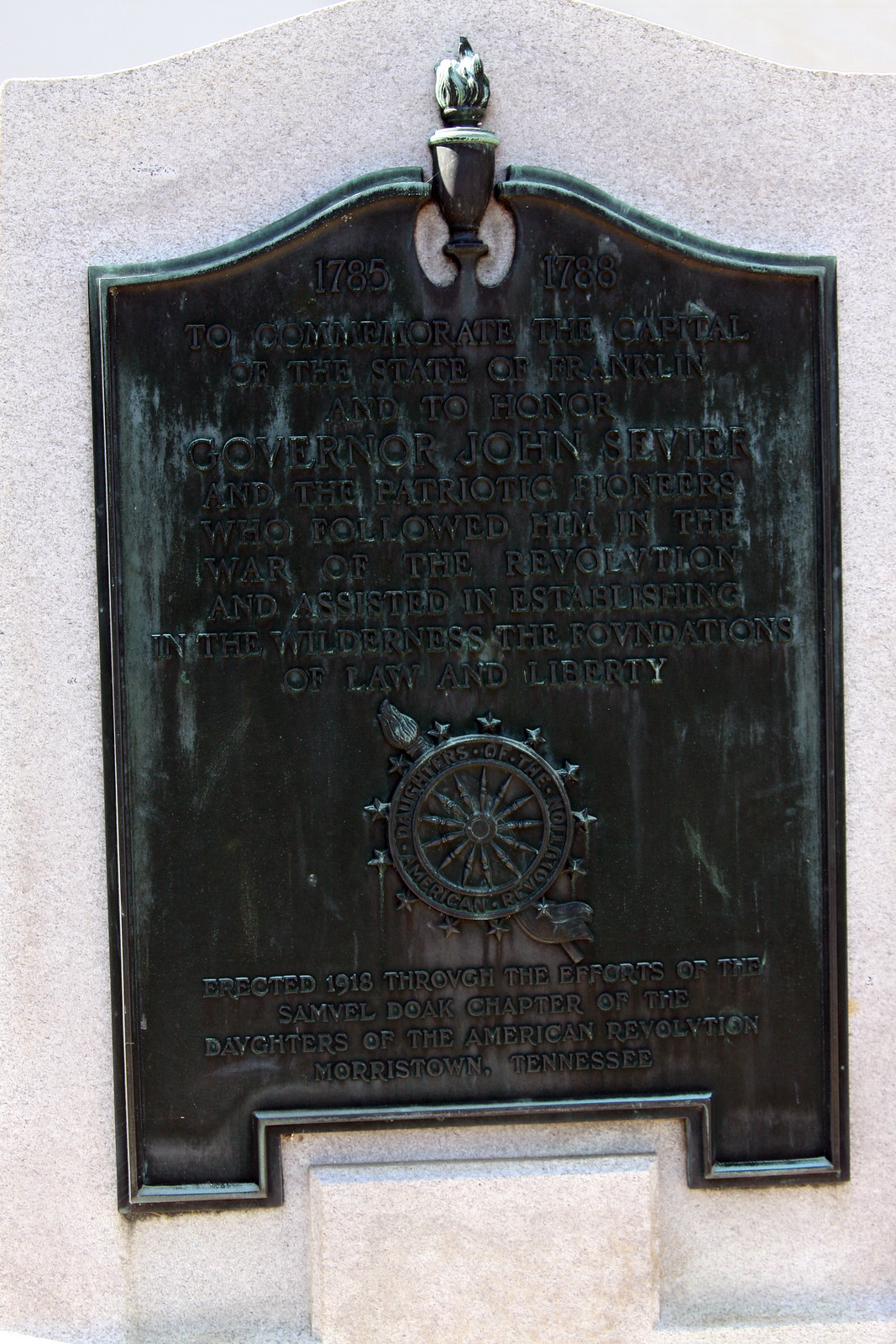This image features a weathered brass plaque mounted on a white, possibly stone, surface, indicating it is located outdoors, likely at a historical site. The central object is a black plaque with an intricate ship steering wheel design, signaling a nautical connection. Although the text on the plaque is partially obscured due to poor lighting and age, several details are discernible. The plaque honors Governor John Sevier and references historical dates, “1785-1788,” to commemorate the capital of the state of Franklin. Additionally, there's mention of the Daughters of the American Revolution, specifically the Samuel Doak chapter from Morristown, Tennessee, with the plaque being erected in 1980. The isolated setting and midday light emphasize the plaque's historical significance and outdoor placement.